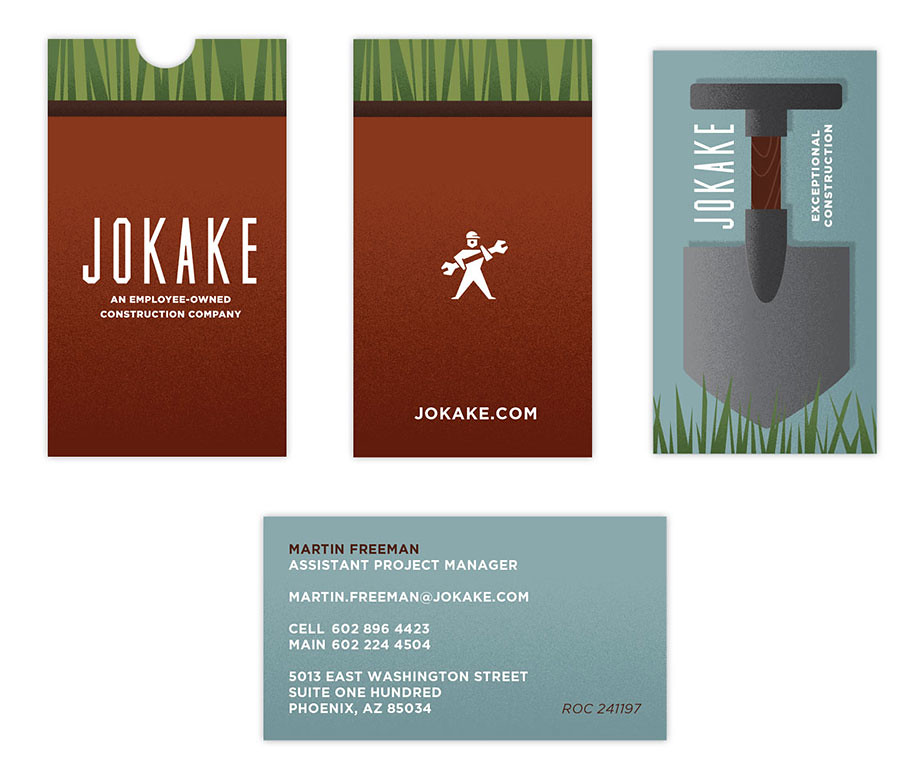The image displays four business cards, showcasing different designs and orientations. The top part of the image features three vertically oriented business cards aligned side by side. The leftmost card bears the name "Joe Cake" with the text "an employee-owned construction company" beneath it, on a brown background with a touch of stylized green grass at the top. The second card, likely the back side of the first, features an illustration of a small man holding a wrench as long as he is, with "JoeCake.com" at the bottom. The third card on the right displays an image of a shovel piercing through grass and is captioned "Joe Cake, exceptional construction."

Below these three cards, centered in the bottom row, lies a horizontally oriented business card. This card belongs to Martin Freeman, titled "assistant project manager," and includes all his contact information. The intricate details and variations in the designs suggest a focus on the construction theme, reinforced by the earthy brown and green color scheme and the tools depicted on the cards.